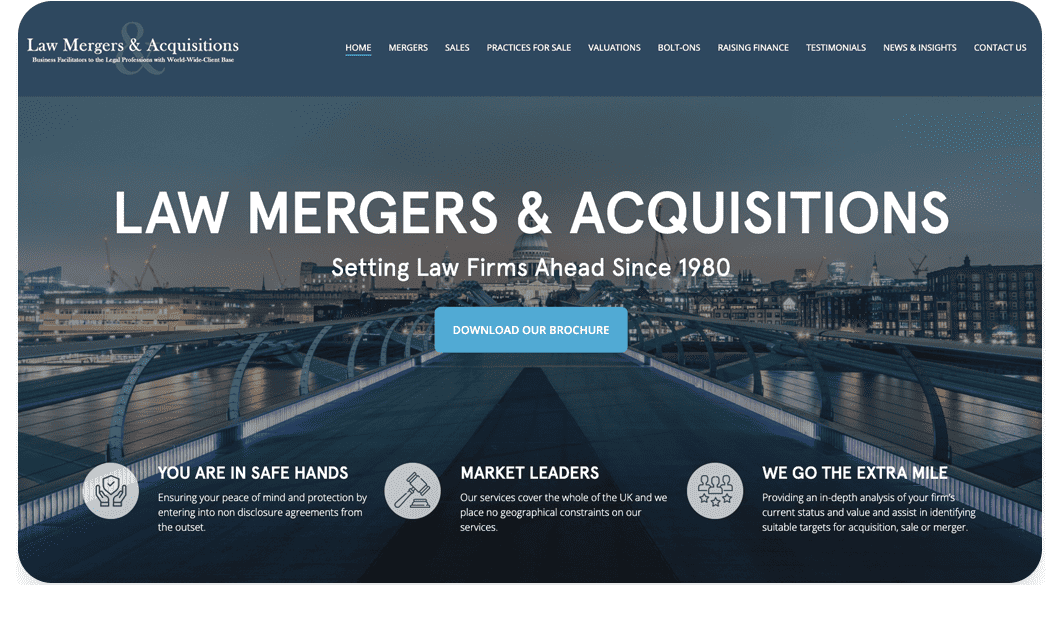The image features a detailed layout for a website dedicated to law mergers and acquisitions. At the top left corner, there is a heading titled "Law Mergers and Acquisitions". Accompanying this on the right is a comprehensive menu listing options such as Home, Mergers, Sales, Practices for Sale, Valuation, Bolt-Ons, Raising Finance, Testimonials, News and Insights, and Contact Us.

Prominently displayed is a scenic photograph of Washington D.C., showing the Congress building in the distance, seemingly as seen from a bridge over a river. Overlaying this image is the text "Law Mergers and Acquisitions," stating that certain law firms have been active since 1980. 

Beneath this, a prominent blue box invites visitors to "Download Our Brochure". Underneath this call to action, on the left side, the text reads, "You're in safe hands," emphasizing the firm's commitment to ensuring client peace of mind and protection through non-disclosure agreements from the outset.

On the right side, the text highlights the firm as "Market Leaders". It states, "Our services cover the whole of the U.K. and we place no geographical constraints on our services. We go the extra mile, providing an in-depth analysis of your firm's current status and value, and assist in..." This suggests a partly detailed yet ongoing description of the firm's comprehensive services.